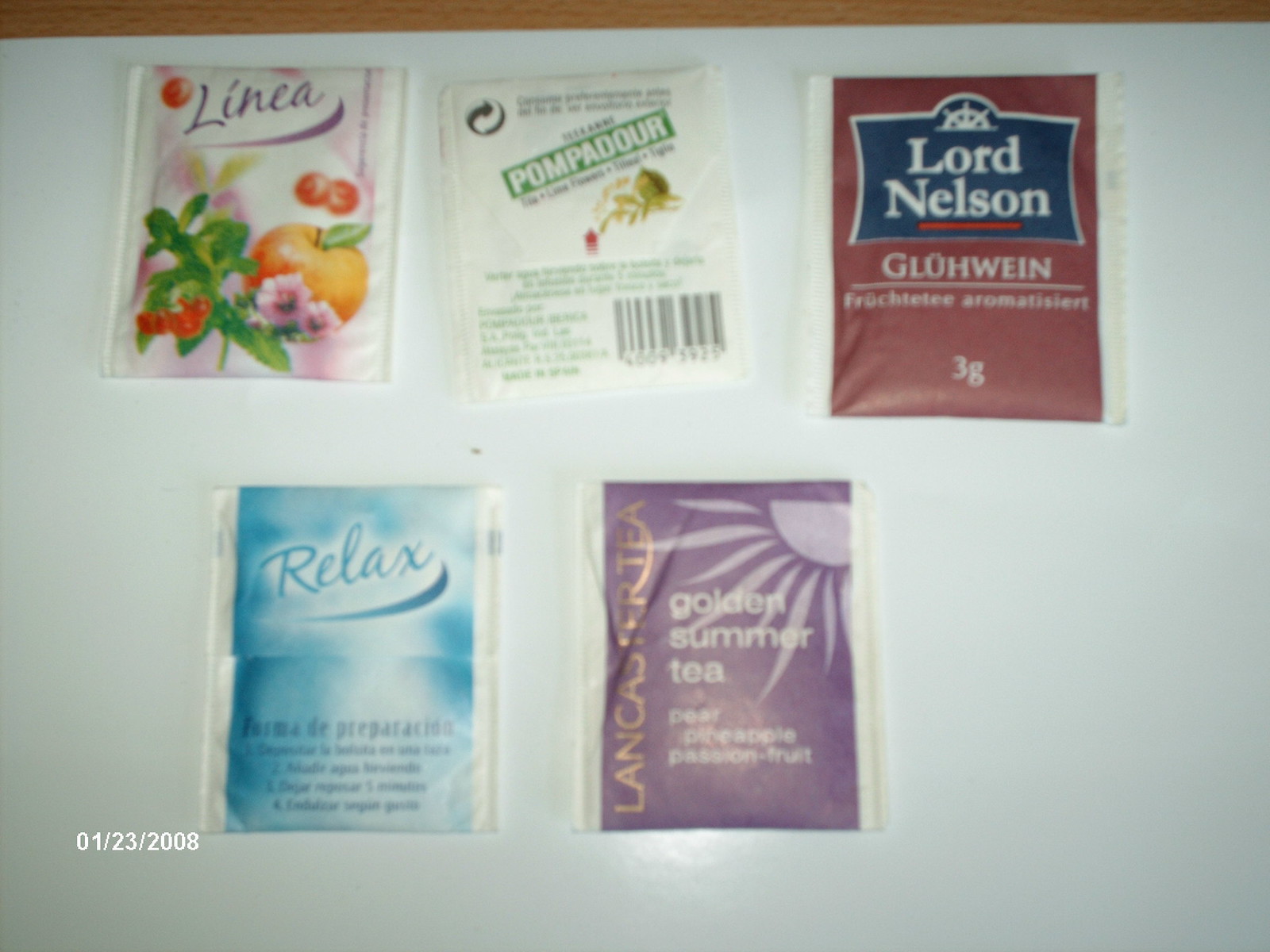This image, dated 01-23-2008 in white text at the bottom left corner, appears to be a somewhat out-of-focus photograph of five different teabag packages arranged on a white piece of paper, with a small strip of a wooden surface peeking through at the very top. The five teabags are from different brands and each has distinct designs and labels:

1. **Top Left:** A teabag with a white background and purple text that reads "Linnea". The design features a prominent red apple surrounded by smaller red fruits, possibly berries or tiny tomatoes, two small purple flowers, and green leaves.

2. **Top Middle:** A white teabag with a green box and white text that says "Pompadour". This package has a prominent barcode in the bottom right corner and some illegible green writing around an image that might be a small nut or fruit.

3. **Top Right:** A teabag with a burgundy-red background, featuring a blue square in the center with white text that says "Lord Nelson". Below this, 'GLÜHWEIN' is written in white text, with additional small German text that's difficult to decipher.

4. **Bottom Left:** A teabag with a tie-dyed blue and white pattern. The bold blue letters with a white glow spell out "Relax" at the top, with some indistinct text below it.

5. **Bottom Right:** A purple teabag, adorned with vertical gold text on the left side that reads "Lancaster Tea". The central white text states "Golden Summer Tea" followed by "pear, pineapple, passion fruit". The background includes a lavender silhouette of a sun.

Each teabag is distinctively branded and colorful, set against the plain white surface with visible wood at the top, emphasizing their varied designs.